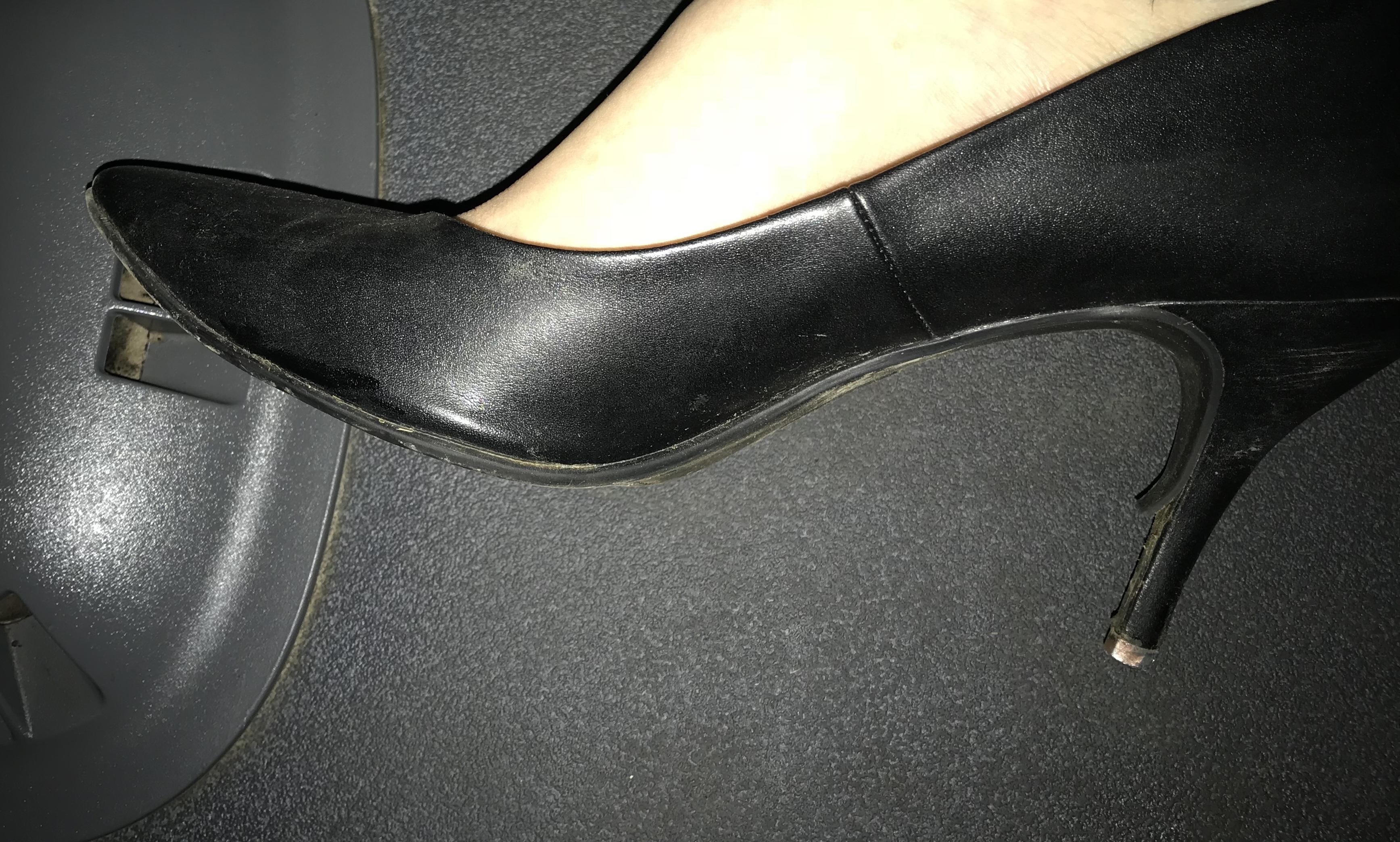This is a detailed, up-close photograph of a woman's high-heeled shoe, highlighting her foot resting sideways within it. The black patent leather shoe, which exhibits significant wear including scratched brown spots and scuffed areas, is set against the backdrop of a car interior, identifiable by its grey fabric and plastic components. The heel is notably damaged, with peeling leather on the inner stack, white scuff marks along the back edge, and a partially detached rubber heel cap. The bright flash used in the photo accentuates the pale complexion of the woman's foot and the worn state of the shoe. The surrounding car interior appears slightly dirty and dusty, emphasizing the neglected state of the setting.